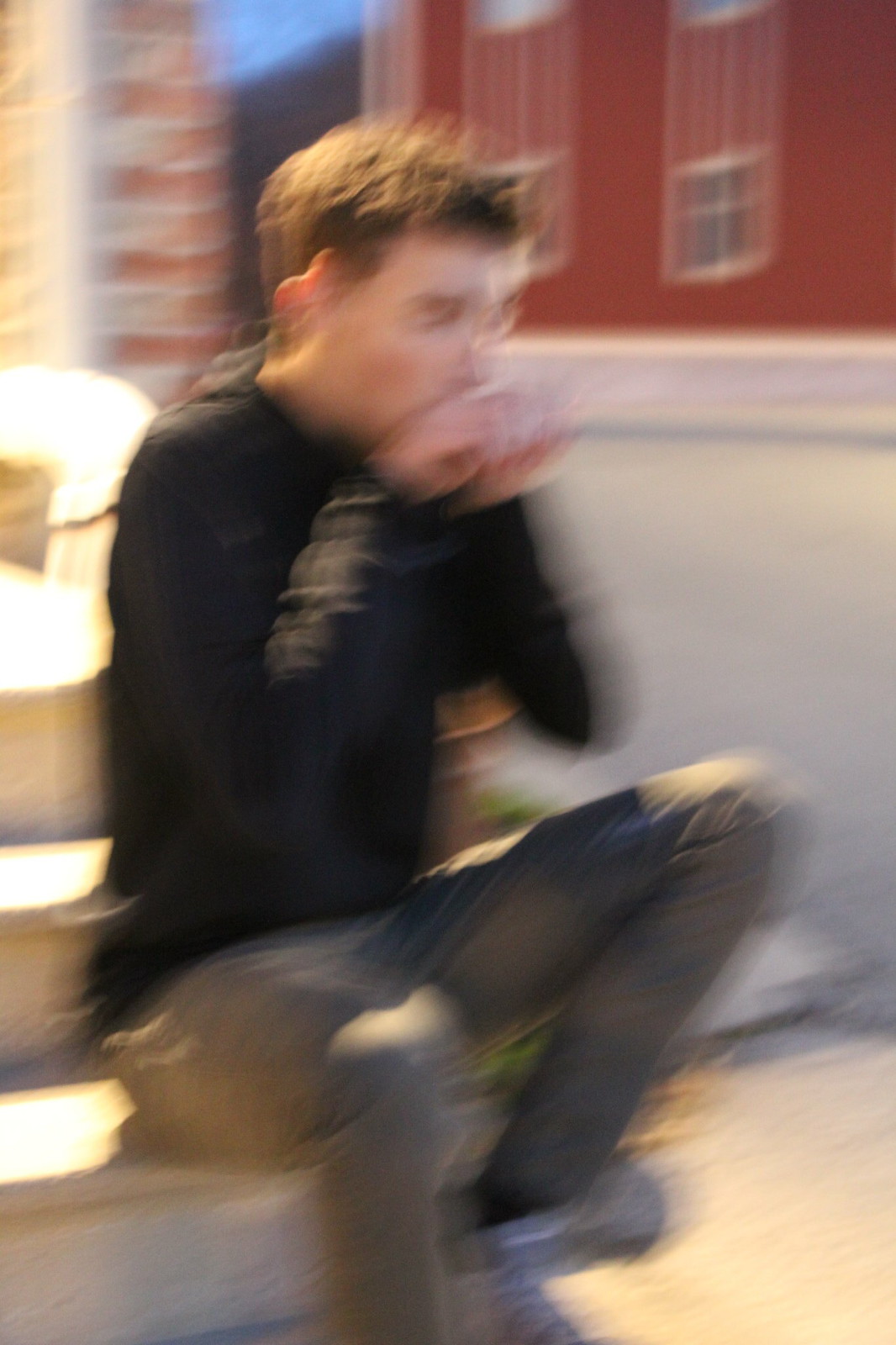This close-up photo, though extremely blurry due to motion sway, captures a white man sitting on the bottom step of a staircase outside a brick house. His short brown hair is styled slightly upward, and he is wearing a black long-sleeve sweater and gray or green chino pants with gray shoes. The man appears to have his hands up to his mouth, potentially eating, smoking, or holding some object, making it hard to determine his exact activity. The scene is illuminated by a fluorescent light from above, suggesting it is nighttime, yet the photo is not particularly dark. In the background, there is a red brick building, a fence, and another red building, hinting at a neighborhood setting.